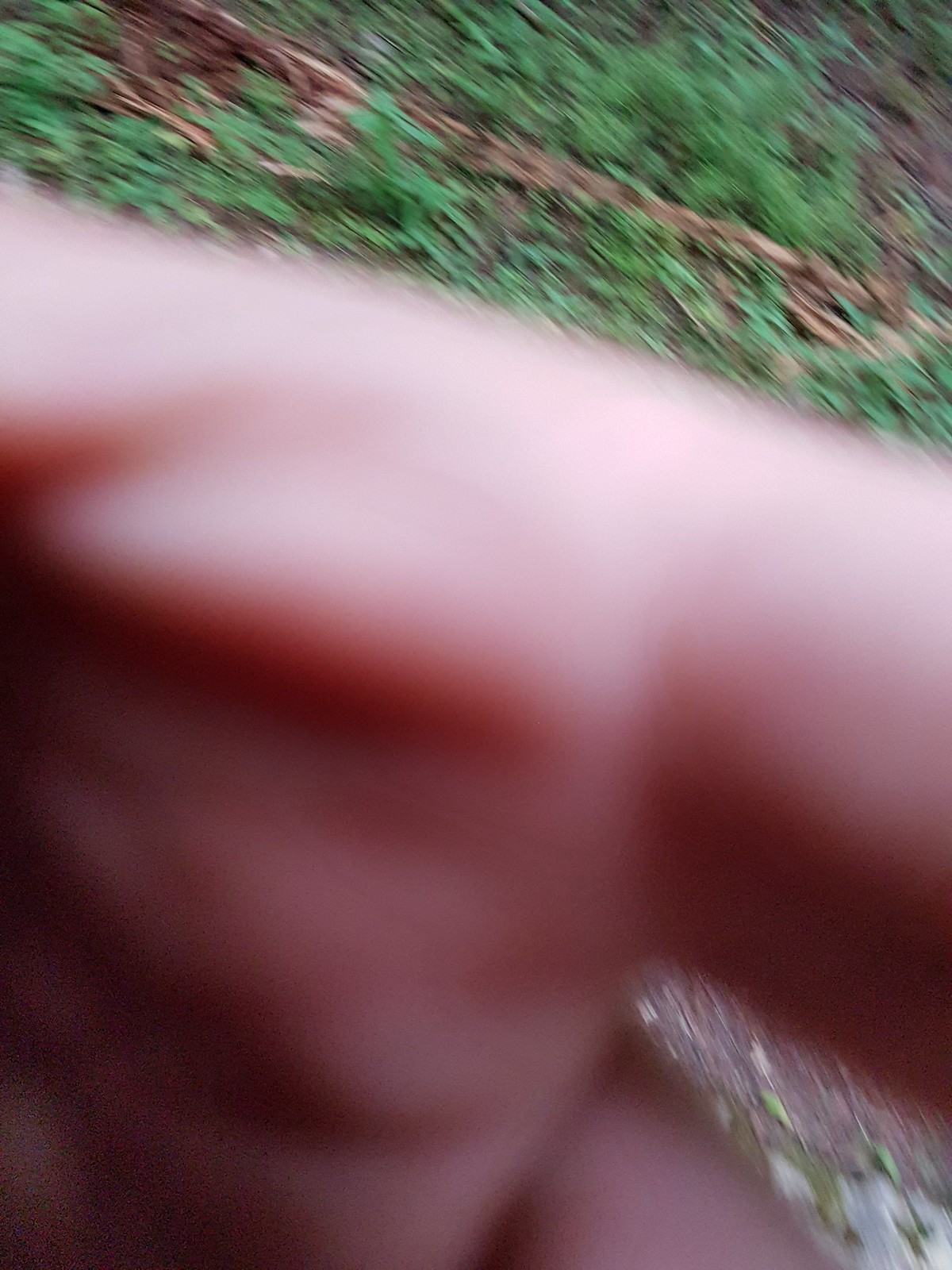An extremely blurry close-up photo shows a white individual's hand covering approximately 70-75% of the camera lens. The person's index finger and part of the thumb are visible, slightly parting to reveal snippets of the background. The background includes patches of green vegetation, such as grass and plants, intermixed with brown branches, stones, and some sand, suggesting a natural, garden-like or park setting. The entire image has a pinkish tint and is heavily blurred, giving the impression of motion or an accidental shot. The green and brown plant life can be seen through the small gap between the fingers, while the lower edge of the image transitions into darkness, making it difficult to discern exact details. The overall effect is a vibrant and chaotic mix of colors and textures, framed by the indistinct shapes of the hand and natural elements.